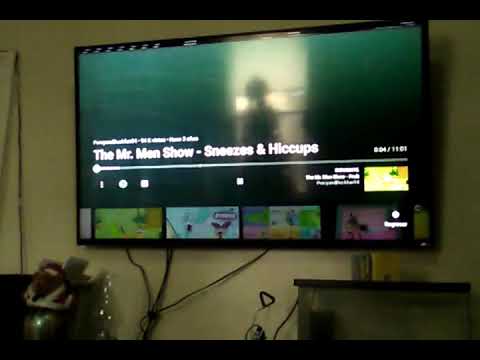The image depicts a dimly lit room with green walls, featuring a large flat-screen TV mounted on the wall. The TV is currently paused on a show titled "The Mr. Men Show: Sneezes and Hiccups," which is displayed on what appears to be a Netflix interface. Below the TV, three cables trail down and disappear behind a stand, which is positioned on the left side. Additionally, there are shelves beneath the TV, possibly on both sides. On the right side of the room, there is what looks like a desk or chest. The TV screen shows a blurry, shadowy figure, set against a bright background, possibly indicating a paused scene. The overall image is slightly blurry, capturing an amateur, home-like quality. The dim lighting suggests an attempt to reduce glare while watching TV, contributing to the cozy, lived-in atmosphere of the room. Various colors such as black, green, blue, pink, yellow, and tan are scattered throughout the scene, adding to the room's character.